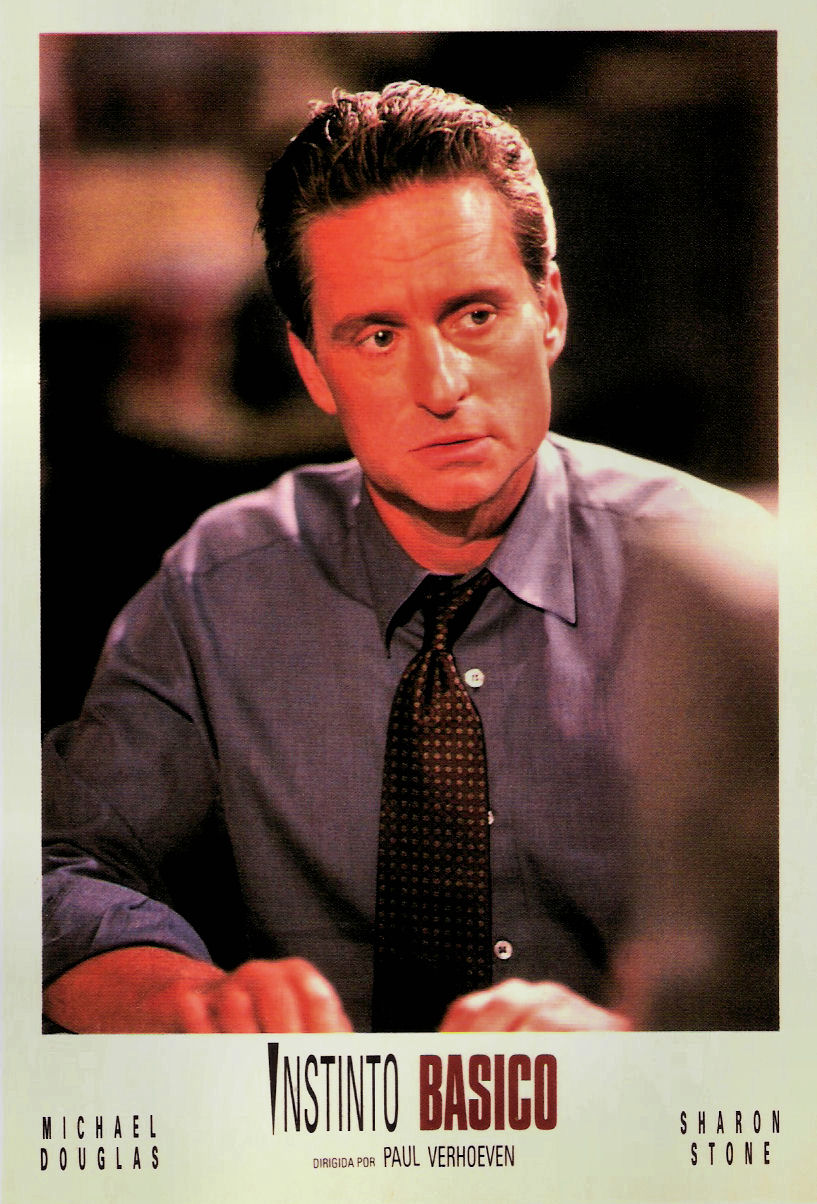The promotional poster is designed as a large beige-framed image of a middle-aged man with slicked-back, dark brown hair, sitting and looking slightly to the right. He is wearing a dark blue button-up shirt with slightly rolled-up sleeves and a black tie adorned with gold polka dots. The man’s head is tilted slightly to the left and his mouth is just barely open, suggesting a moment captured from a film. The background is blurred, focusing attention on the man’s contemplative expression. At the bottom of the photograph, in thin black text, it reads "Instinto," followed by "Basico" in bold red font. Below this, in smaller black font, it states "Dirigida por Paul Verhoeven." In the bottom left corner, it prominently features the name "Michael Douglas" in all caps, and in the bottom right corner, it similarly displays "Sharon Stone" in all caps.